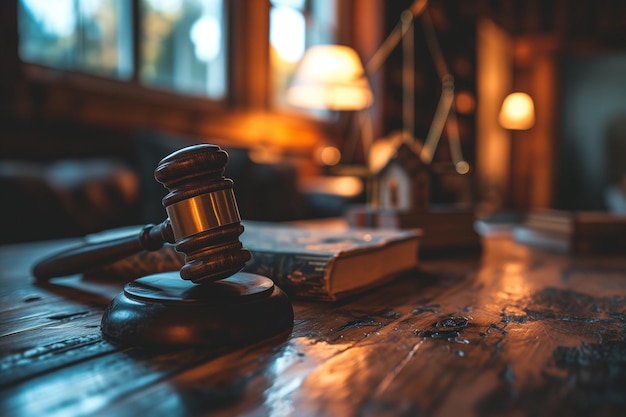The photograph captures a richly detailed, ambient-lit classical study. The immediate foreground features a prominently positioned gavel resting on a stand, the head pointing to the right, situated on an aged, rough pine board table stained in a deep reddish-brown hue. Adjacent to the gavel lies a dark-colored, worn-edged book. The background blurs into soft focus, revealing hints of additional elements: faint images of windows, lamps, more books, and what seems to be a model house. A distinctive grandfather clock and a chair can be discerned amidst the out-of-focus scenery. The light from the lamps softly illuminates the worn table, adding character to the setting. The absence of visible lettering, people, or animals in the photograph directs all attention to the tactile and historic elements of the gavel and the sophisticated, book-lined backdrop, imparting an air of solemnity and purpose to the space.